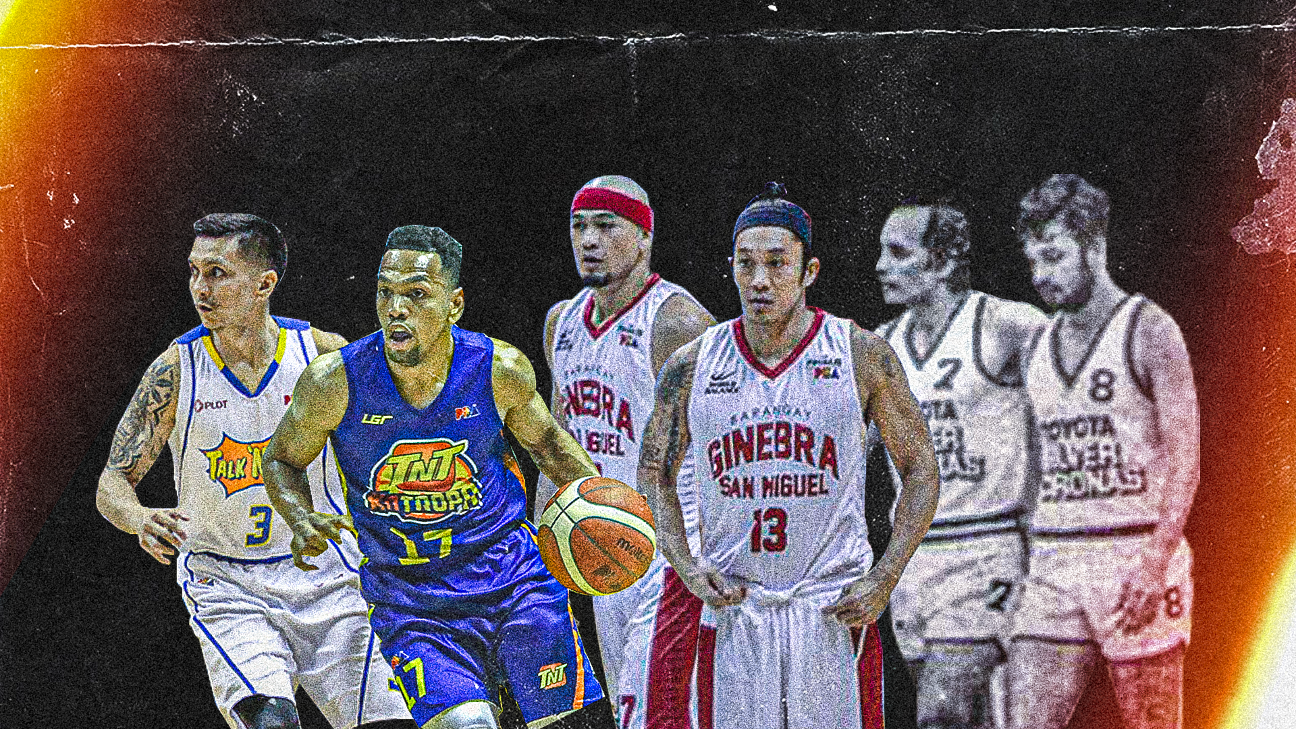The image is an aged and slightly discolored photograph showcasing six basketball players from various teams. On the far left, there is a player in a white jersey with blue and yellow stripes, featuring a blue number 3 and a PLDT logo. Next to him, a player in a blue uniform, adorned with a TNT logo, dribbles an orange and white basketball with his left hand; his jersey has the yellow number 17. Positioned center-right are two players from the same team—they wear Ginebra San Miguel jerseys, which are white with dark red lettering and red collars, and white shorts with red stripes. The visible details on their uniforms include partial letters spelling "Ginebra" and the numbers 12 and 13. In the background, there are two black and white players standing out due to the monochrome treatment; their jerseys display the Toyota logo and have numbers 7 and 8. The players in Ginebra uniforms appear to be Filipino, adding a cultural dimension to the scene. The photograph's age is further emphasized by a crease across the top and areas of discoloration in the top corners.